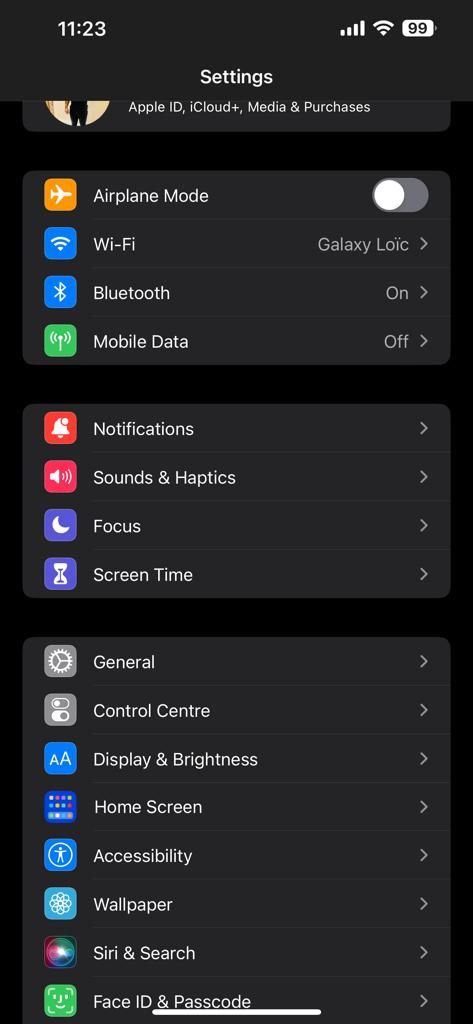This screenshot captures a smartphone display with a solid black background. In the upper-left corner, the time is shown as 11:23. The upper-right corner indicates full Wi-Fi signal strength with 5 bars and a battery level at 99%. 

Dominating the center of the screen is the heading “Settings” in white text, followed by “Apple ID, iCloud, Media & Purchases.” Below, a series of options are listed:

1. **Airplane Mode** 
2. **Wi-Fi** - Connected to "Galaxy Loic"
3. **Bluetooth** - On
4. **Mobile Data** - Off
5. **Notifications** - Accompanied by a red box with a small bell icon.
6. **Sounds & Haptics** - Accompanied by a red square with a speaker icon.
7. **Focus** - Accompanied by a blue box with a moon icon.
8. **Screen Time** - Accompanied by a blue box with a timer icon.
   
Further down the list are:

1. **General**
2. **Control Center**
3. **Display & Brightness**
4. **Home Screen**
5. **Accessibility** - Accompanied by a blue box with a person in a circle icon.
6. **Wallpaper** - Accompanied by a blue box with a snowflake-like icon.
7. **Siri & Search**
8. **Face ID & Passcode**

The image is a precise capture of the settings screen of an iOS device, meticulously detailing the various menu options available.